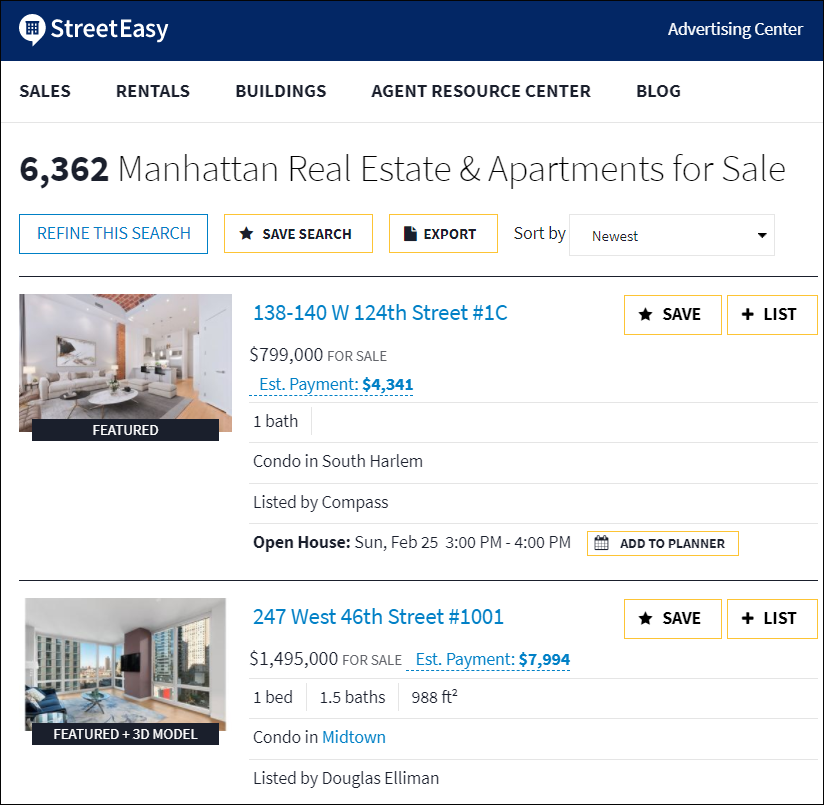**Caption:**

This image is a screenshot of a StreetEasy webpage. The top banner is dark blue with white text, displaying "StreetEasy" on the left, with capitalized "S" and "E," and "Advertising Center" on the right. Below this banner, there are navigation links in black font on a white background, all in capital letters: "SALES," "RENTALS," "BUILDINGS," "AGENT RESOURCE CENTER," and "BLOG." A thin gray line separates the navigation bar from the content below.

The main content begins with bold text displaying "6,362" in black, followed by "Manhattan Real Estate and Apartments for Sale" in gray. Below this, three buttons are aligned horizontally on the left: the first button is blue, outlined in blue, and reads "REFINE THIS SEARCH" in capital letters; the second button is gold with black text, reading "SAVE SEARCH" and featuring a star icon on the left; the third button is also gold with black text, reading "EXPORT" alongside a bookmark page icon.

To the right of these buttons, there is a sorting option allowing the user to sort listings. The sorting box is gray-outlined with the word "NEWEST" and a pull-down arrow.

The lower section showcases two apartment listings. The first listing is for an apartment on 124th Street, priced at $800,000, with the address in blue font. The second listing is for an apartment on 46th Street, priced at $1.495 million, and described as having one bedroom and one and a half bathrooms.